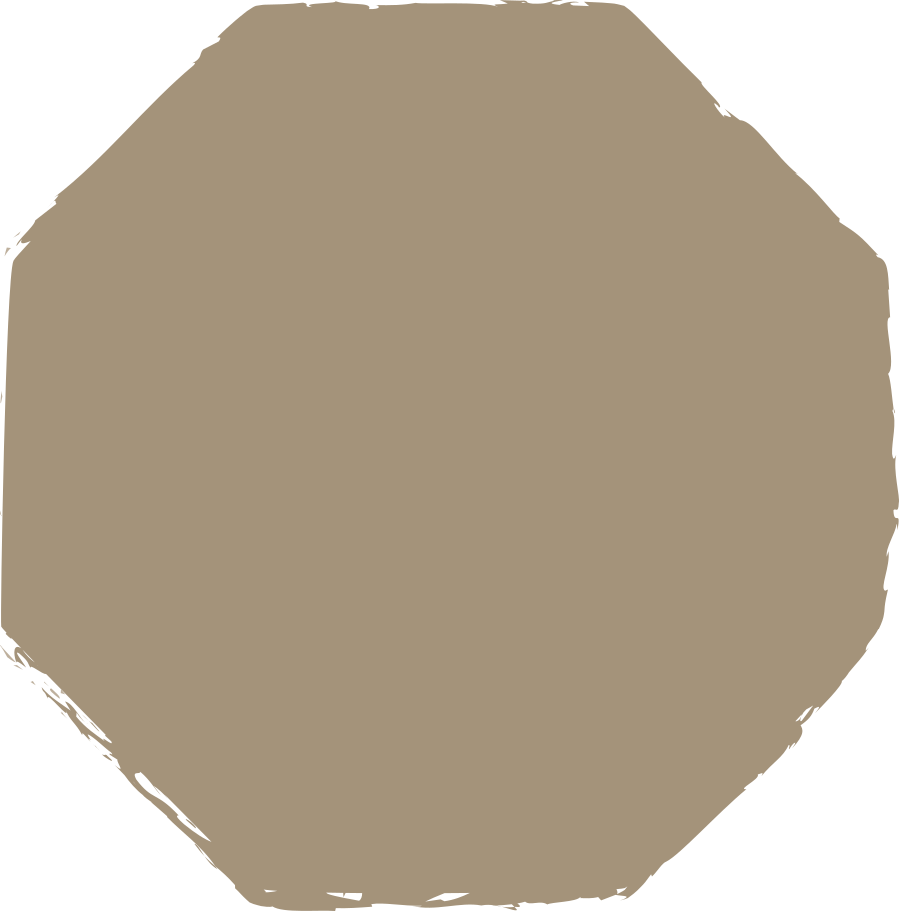This detailed image depicts an abstract representation of an octagonal shape, heavily leaning towards an octagonal outline despite its imprecise and jagged edges. The octagon is primarily filled with a light brown or grayish clay color that occasionally bleeds beyond its borders, giving it a somewhat handwritten appearance. Notably, the bottom left edge, in particular, appears more distorted and splashed, adding to its irregularity. The background is stark white, providing a stark contrast that further highlights the roughness of the octagonal figure. Despite the lack of any text, the overall design suggests a large, simplistic sign with a hand-painted aesthetic.